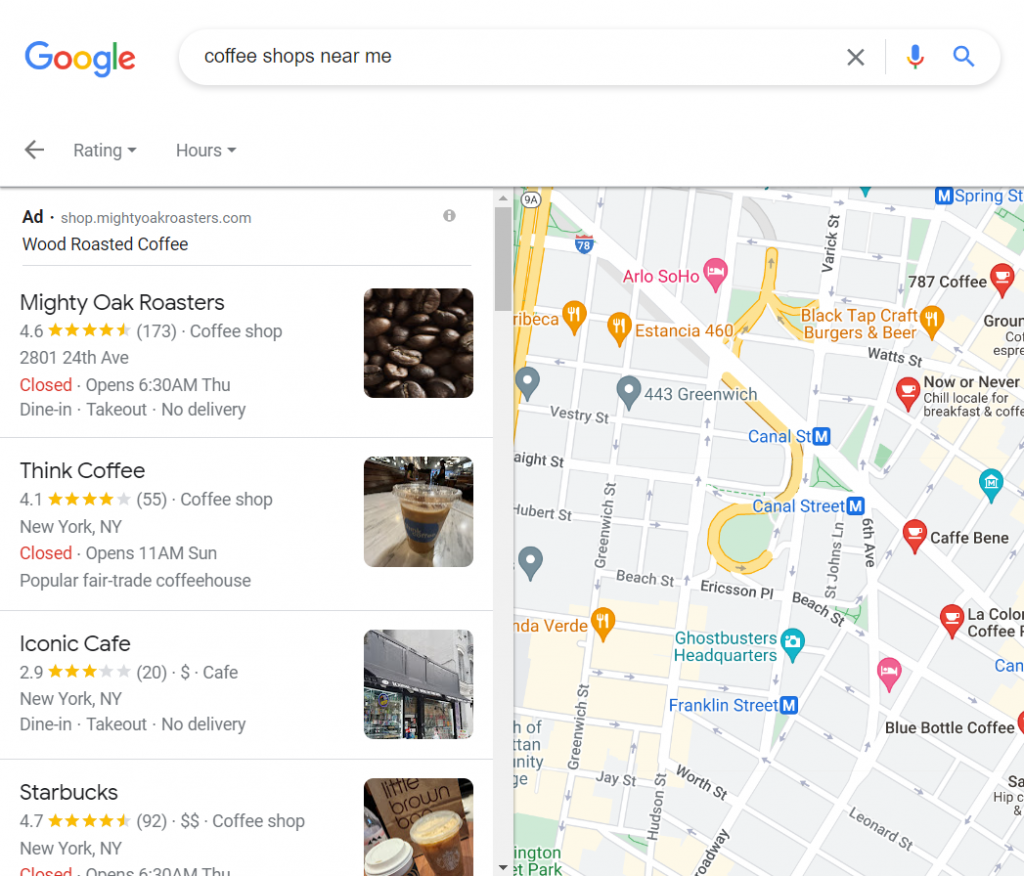A Google search page is displayed with the Google logo prominently featured in the top left corner, exhibiting its iconic multicolored letters: blue, red, yellow, blue, green, and red. In the search bar, the query "coffee shops near me" is entered. Adjacent to the search bar, several familiar icons are visible: a gray 'X' button, a microphone icon, and a magnifying glass icon.

Directly below the search bar, a list of nearby coffee shops is presented. The first entry is for Mighty Oaks Roasters, which boasts a rating of 4.6 stars based on 173 reviews. It is located at 2801 24th Ave. While currently closed, it will open on Thursday at 6:30 a.m., offering options for dine-in and take-out, though delivery is not available.

The second entry is Think Coffee, holding a 4.1-star rating from 55 reviews. This popular fair trade coffeehouse is situated in New York, New York and is currently closed, with an opening time of 11:00 a.m. on Sunday.

Lastly, Iconic Cafe is listed with a modest 2.9-star rating from 20 reviews and a single dollar sign indicating its price range. Also located in New York, NY, this cafe provides dine-in and take-out services but does not offer delivery.